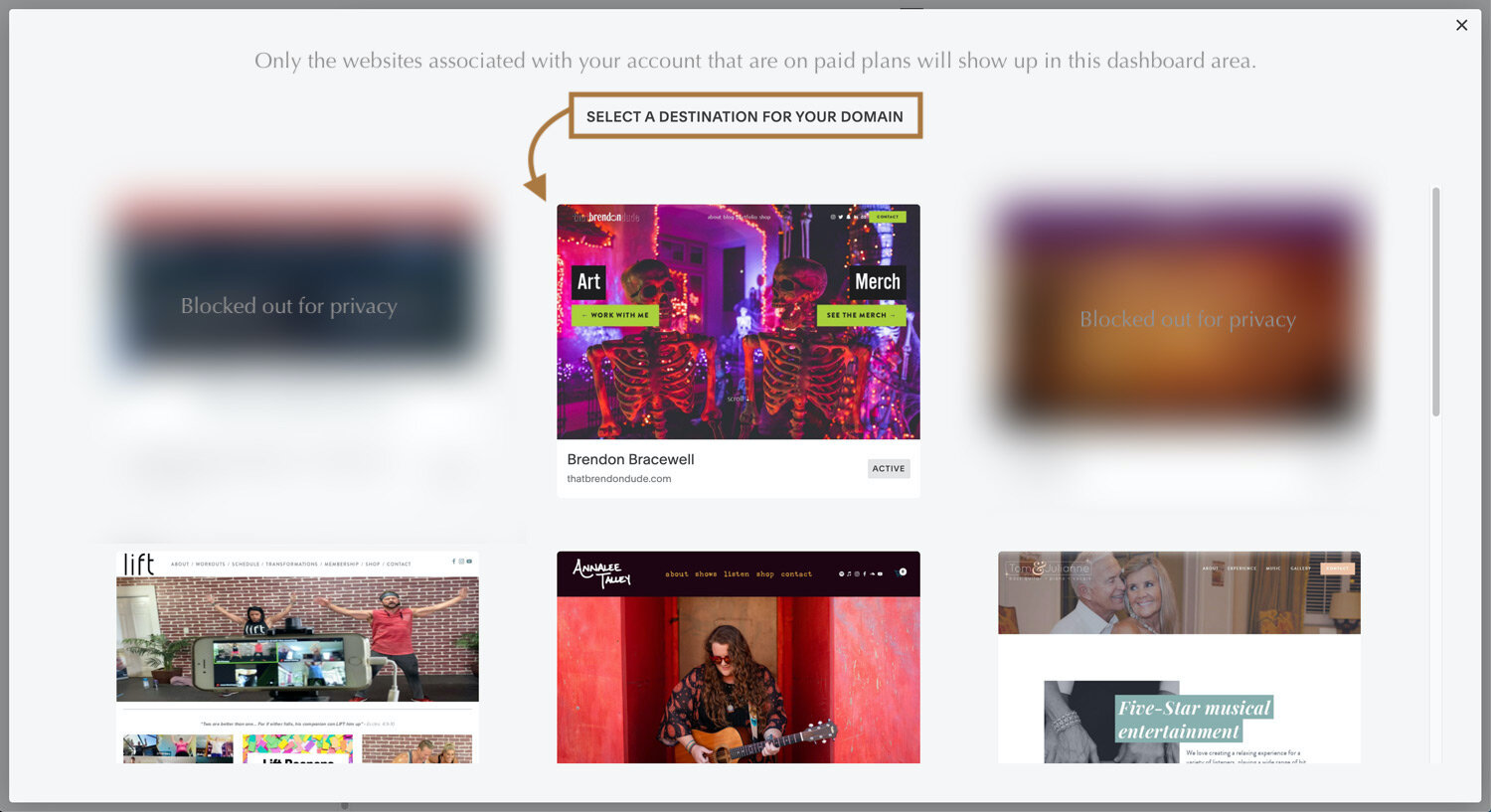The dashboard screen displays a message indicating that only the websites associated with your account on paid plans will be visible in this area. The interface showcases six images, two of which are intentionally blurred and marked as "blocked out for privacy." The remaining visible images are eclectic: one features a person playing a guitar, while another displays two skeletons in a setup that appears curated. Above the visuals, a text box prompts the user to "select a destination for your domain," suggesting functionality for managing multiple websites. The predominant background color is white, and the layout implies there's more content accessible through scrolling.